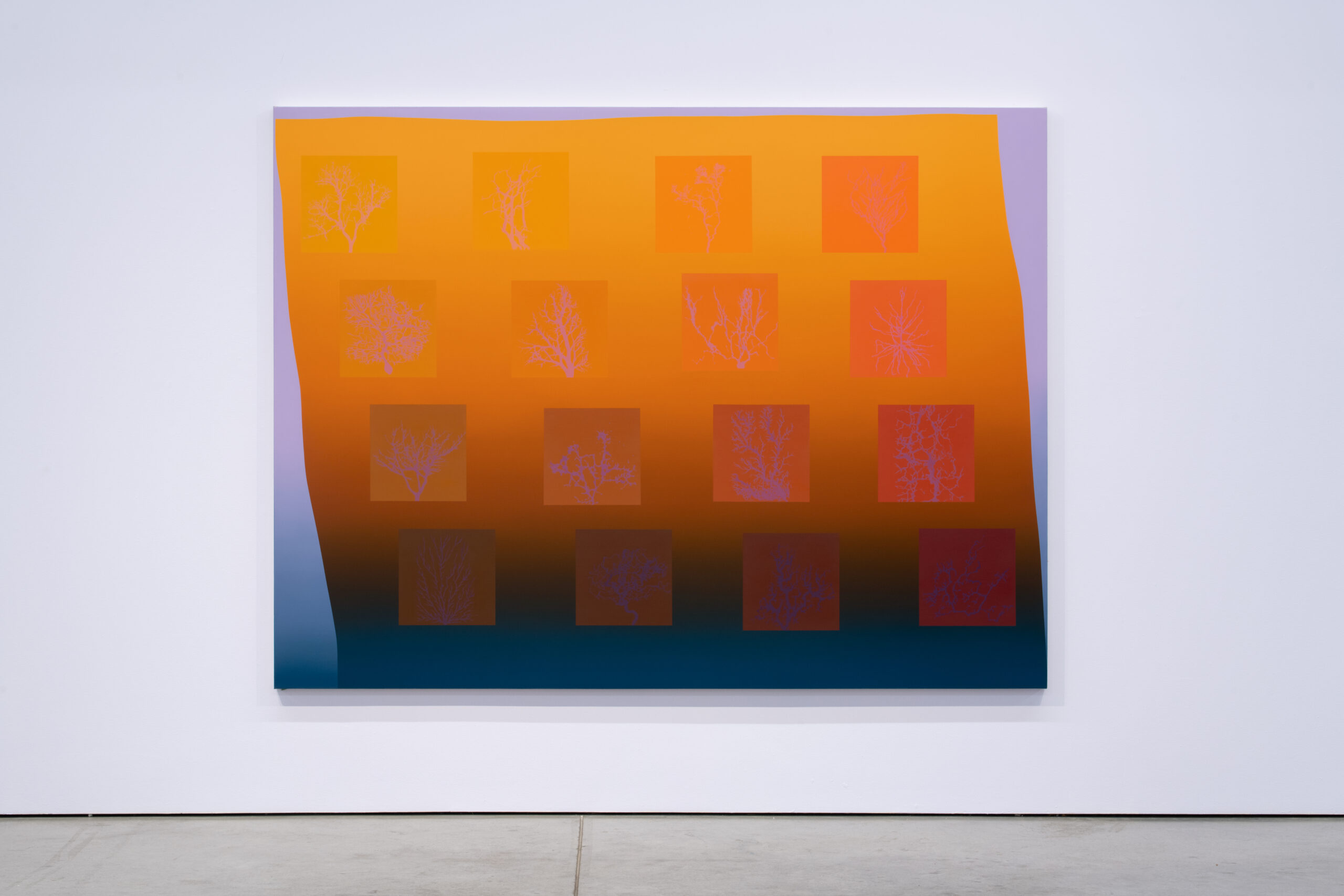The image depicts a modern abstract art piece, displayed on a white wall within a museum, with white concrete flooring. The artwork is a large, unframed rectangular canvas, comprising a striking grid of sixteen squares (arranged 4x4) with spaces in between. The overall image features a compelling ombre gradient that transitions from bright orange at the top, through shades of red and rust, to a deeper brownish-blue at the bottom. Each square within the grid showcases its own gradient, aligned diagonally and marked with purplish scribbles, adding a dynamic texture to the piece. The entire composition appears slightly tilted, enhancing the abstract quality and creating a sense of movement. This visually engaging artwork blends hues of purple at the edges, contributing to its mesmerizing and almost surreal aesthetic.